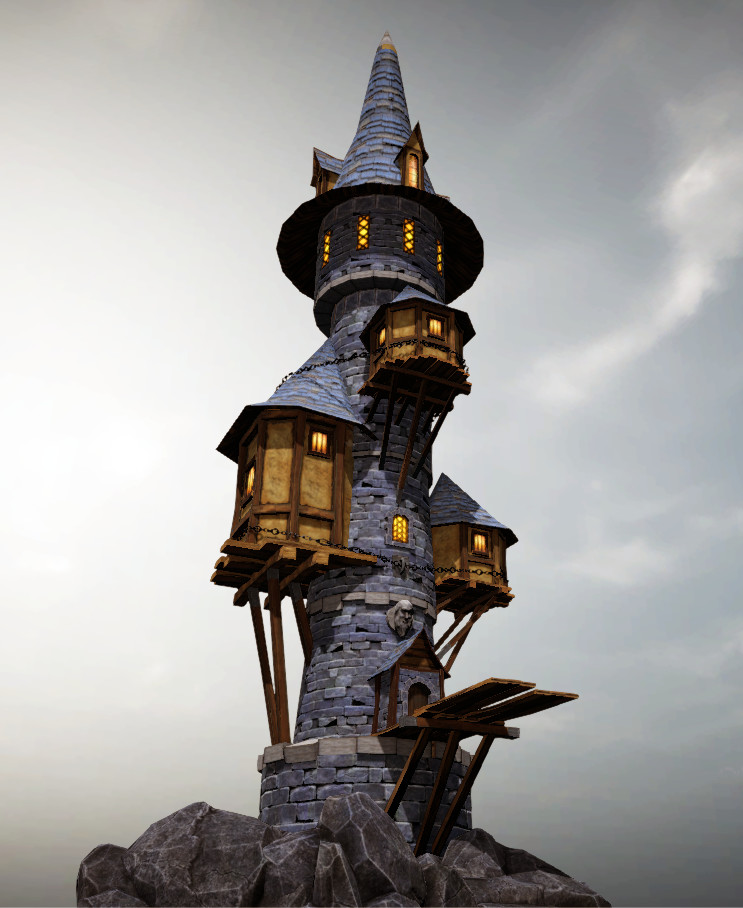This image depicts a towering, slender, and somewhat eerie castle set against a light grayish-blue sky with sparse white clouds. The base of the castle is anchored in a jagged rock formation, a mix of light and dark grays. The castle extends upward for five intricate floors, each level becoming slightly narrower as it ascends.

The ground level features a blue concrete facade with silver concrete trim. A small brown door, framed in blue, leads to a wooden plank walkway supported by three wooden braces, giving it the appearance of a gangplank.

On the next level, a wooden hut protrudes from the left side of the castle, characterized by its brown walls and gray roof. The hut has two windows, one on the front and one on the side, both lit up. This level also features a singular light at its center, glowing against the dark bluish-gray stone.

The third level houses another small wooden extension on the right side, similar in structure to the previous hut but with one window. The main structure on this level is dark gray with lighter brick borders, connected by chains to similar extensions.

Ascending further, the fourth level mimics the gray stone pattern and features yet another hut with yellow-lit windows both on the left and front sides. The topmost level rounds off with an observation-like steeple topped by a witch's hat-shaped roof. This pointed peak is blue, and just below it, four windows emit a warm yellow light, adding to the castle's mystical aura.

The entire scene resembles something plucked from the pages of a fantasy novel, akin to the whimsical spires found in the works of J.K. Rowling or J.R.R. Tolkien.